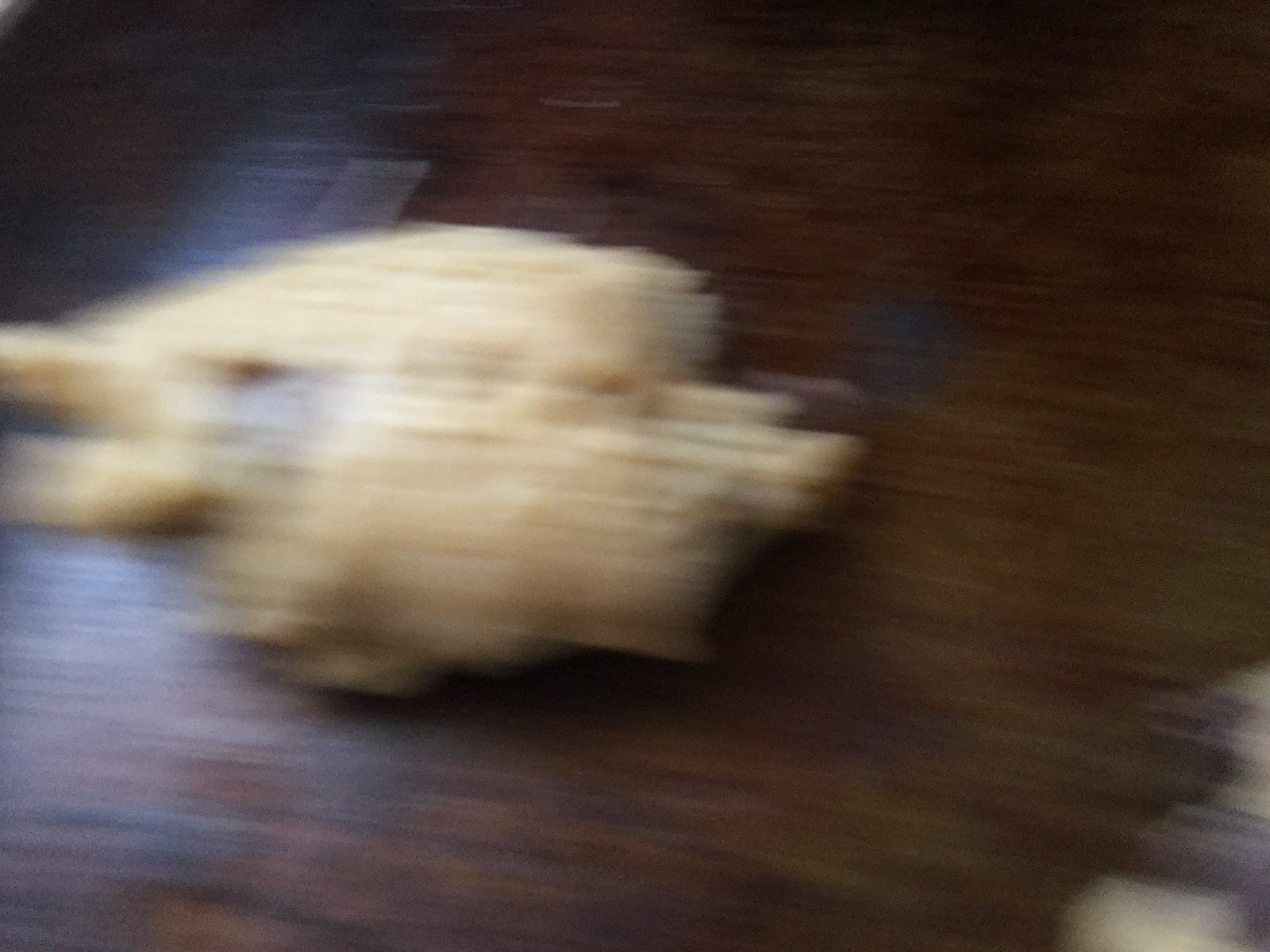The photograph depicts a highly blurred scene featuring a yellow, non-uniform textured object on a reddish-brown and blue ground. The object, reminiscent of a chicken in shape, displays varied textures and is accompanied by another similar yellow blurry form marked with blue in the bottom right corner. The overall image suggests motion, as evidenced by horizontal blur lines indicative of the camera moving left to right. In the background, there's a light source directed towards the left side, contributing to the uneven lighting. The ground is primarily brown with streaks of blue, resembling a marbled surface. The combination of colors and blurred elements creates an indistinct but dynamic image, dominated by the contrasting lighter yellow objects against the darker brown and blue backdrop.